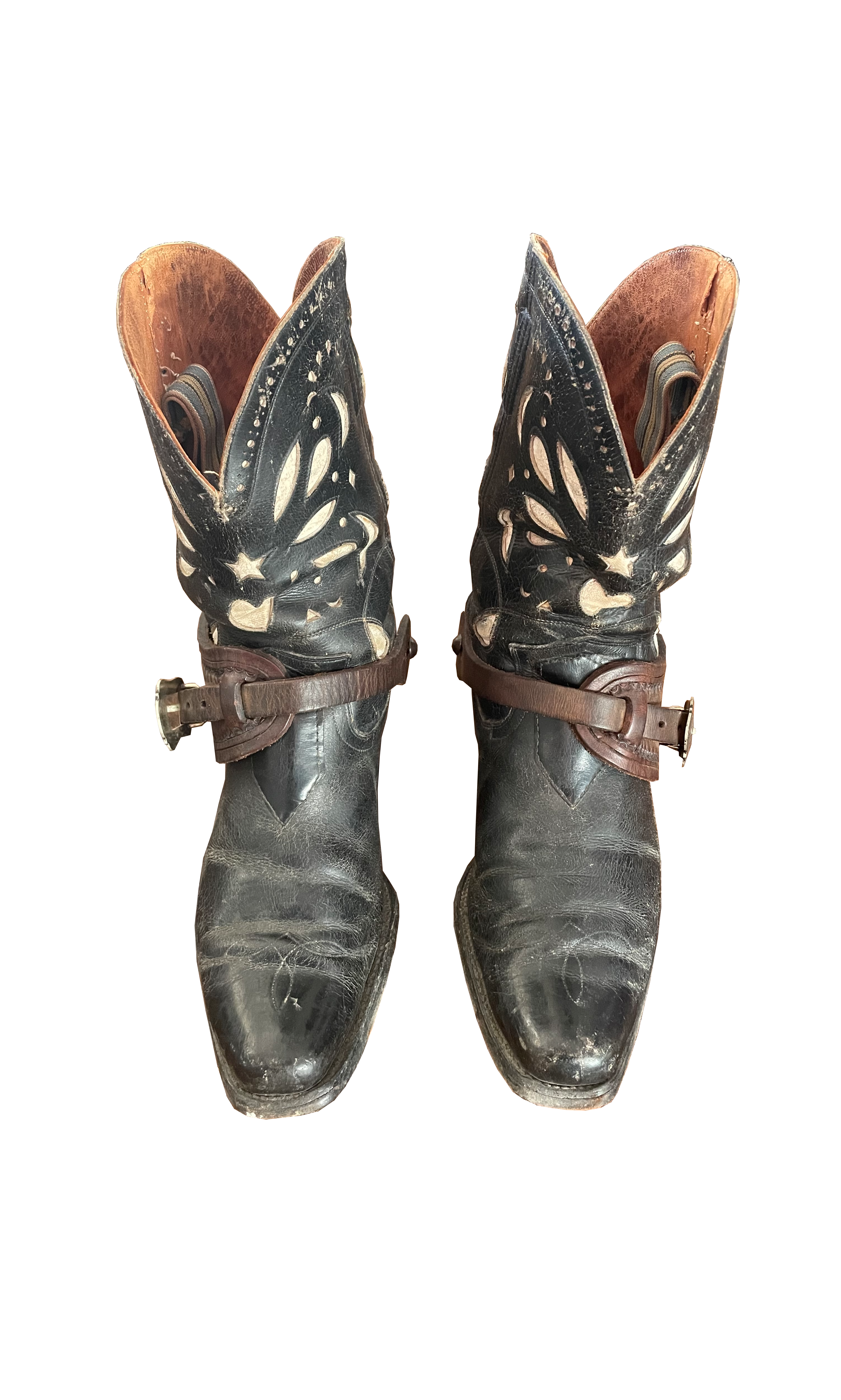The image is a vertical product photograph of a pair of well-worn cowboy boots, displayed against a plain white background, making them appear to float in an empty void. The boots, which were originally black, now exhibit a heavily faded and cracked grayish-black leather, showcasing numerous creases, wrinkles, and indents from extensive use. Distinctive, intricate cut-out designs in the leather, resembling hearts, teardrops, and star-like shapes, reveal an off-white layer beneath. These designs give the impression of butterfly wings with a star at the center. The shafts of the boots feature brown suede interiors with light gray and pink-strapped pull tabs folded down. Around the ankle sections, brown leather straps with bronze-colored buckles are secured, most likely to attach the black spurs that are strapped onto the back of the boots. The toes of the boots are distinctly squared, reinforcing their rugged and timeworn appearance.